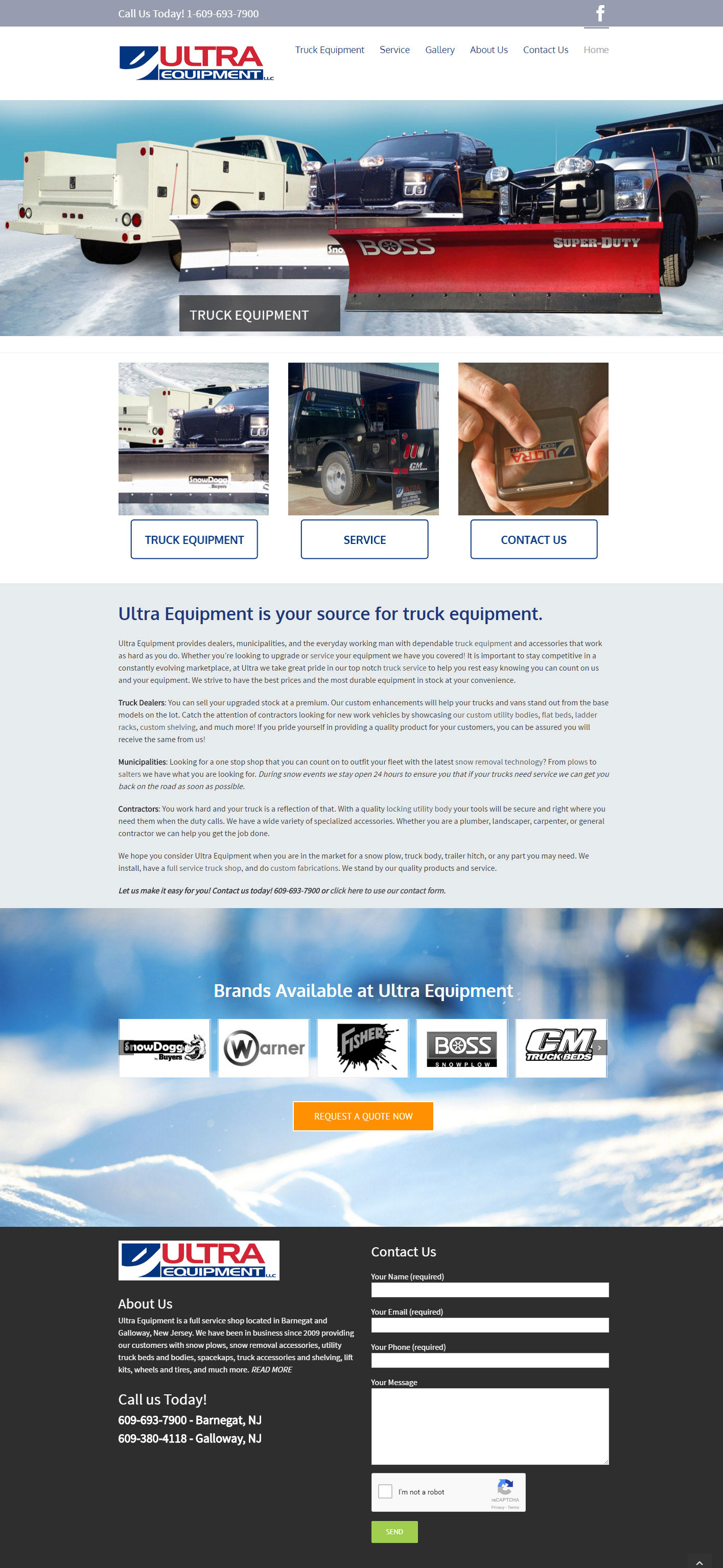The image depicts a zoomed-out view of a website. At the top of the page, "Ultra" is prominently displayed in red text against a gray background. To the right of "Ultra" are six small gray category labels. 

Below this header section, there are images of three trucks. The first truck, positioned on the left, features a red plow. The middle truck has a gray plow attached, and the third truck, seen from the rear, is white. 

Underneath the truck images, there are three square images, each paired with an option button. 

Following this section is a light gray rectangular background containing paragraphs of informational text. Heading this section is the blue text: "Ultra Equipment is your source for truck equipment." 

Directly below, five white squares each contain an emblem or logo. A small, light orange rectangle is below these emblems, featuring some white text against a blue and white, snowy-themed background.

At the very bottom of the page, against a dark gray background, the "Ultra" name is repeated. To the right of this footer are several fields for inputting information, ending with a green submit button.